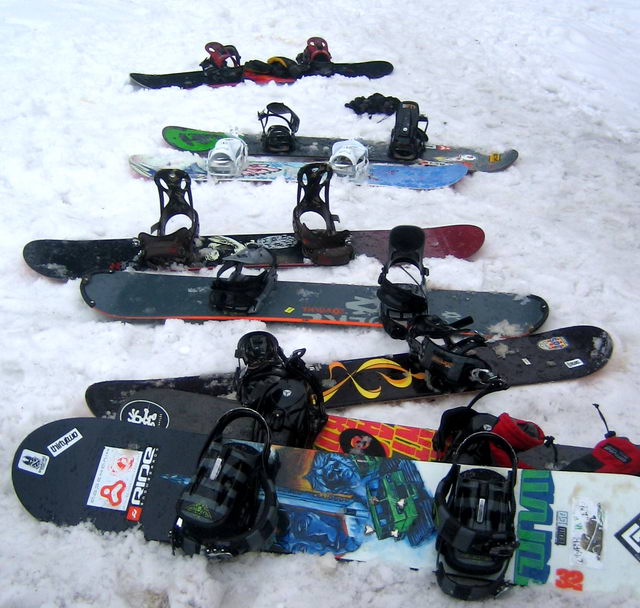This overhead image captures several snowboards laid out in the snow, with the snow appearing slightly gray in the far right corner. The scene features eight snowboards, each with unique and stylish graphic designs, including logos likely from snowboarding or clothing companies. The snowboards are equipped with foot latches for securing the snowboarder's feet. Starting from the front, the first snowboard is black with blue figures and a green box. The second snowboard, partially covered by the first, features black with red and yellow accents. The third is black with wavy yellow patterns. The fourth snowboard has a black base with a red outline, followed by a fifth black snowboard with purple edges. The lineup also includes a blue and gray snowboard next to each other, ending with a fully black snowboard at a distance. The snow beneath these snowboards has been visibly disturbed from activity, suggesting this is an active area on a mountain, despite the zoomed-in focus.